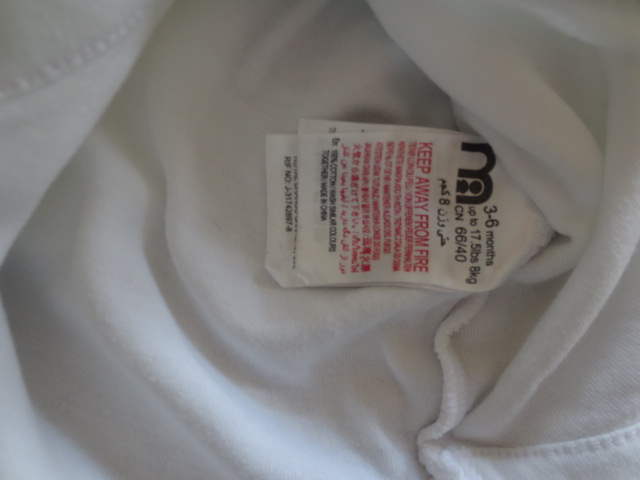The image showcases a white garment resembling a soft sweatshirt material, likely designed for a baby. The interior tag, which is visible, indicates the size range of 3 to 6 months. Prominently displayed in red lettering on the back of the garment is the warning message "KEEP AWAY FROM FIRE." There is also a visible letter "M," presumably the logo of the brand. Beneath the warning message, additional red text is present, though it appears blurred and unreadable. The detailed stitching inside suggests that this item might be a towel or bathrobe for babies, complete with a hood for added warmth and comfort.